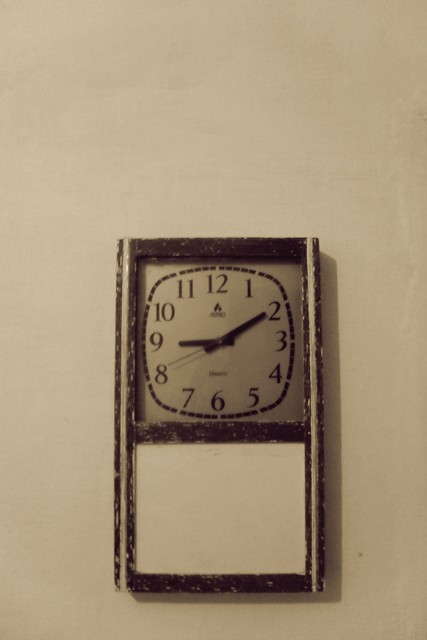This detailed photograph captures a vintage clock mounted on a white plaster wall. The image, though primarily black and white, carries a distinctive brownish tint, giving it a sepia feel. The clock itself is vertically oriented and rectangular, housed in a worn, wooden frame that appears weathered with age. The clock's face is light-colored, almost gray, and is designed with a dashed outline forming a square with heavily rounded corners. 

The hour markers are dark, either in black or deep brown, matching the thick, dark hour and minute hands. In contrast, the second hand is slender and needle-like. Beneath the number 12 and just above the number 6, faint inscriptions are visible but illegible. A shadow cast by the clock adds depth, falling on the wall behind and underneath the clock.

To the right of the clock, a faintly visible, repaired crack in the plaster hints at the wall's history. Below the clock, a horizontal wooden strip contrasts with the white space, which transitions into what seems to be an undisturbed whiteboard area. This juxtaposition of elements adds to the composition's nostalgic ambiance.